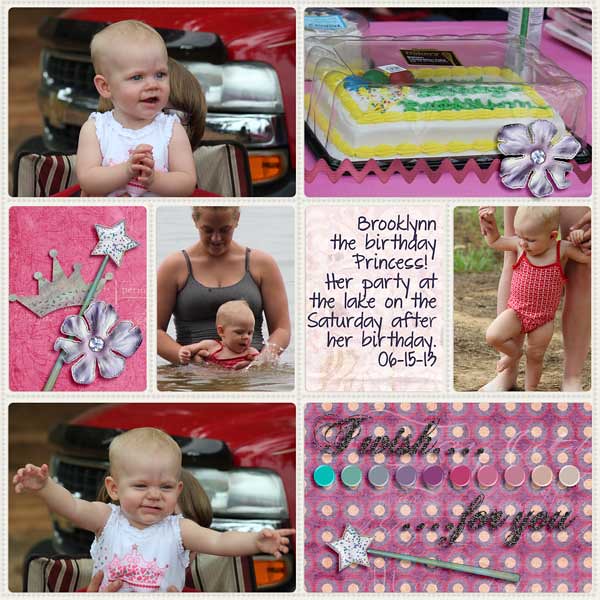This is a detailed, full-color collage composed of several photographs with a light gray border that separates them. The top row features two photographs; on the upper left, a charming little baby girl with very light blonde hair, about one year old, wearing a white top, and smiling with her hands together. Behind her, there’s a red truck. To the right, there’s a vibrant image of a white and yellow birthday cake decorated with green writing, housed in a plastic container. 

The middle section consists of four photos: starting from the left, there is a decorative setup featuring a crown, a flower, and a magic wand with a star on top. Next to it is a touching scene of the baby in the water with her mother, who is wearing a gray swimsuit. The third image is text in right-aligned black, stating, "Brooklyn, the birthday princess. Her party at the lake on Saturday after her birthday, 06-15-13." The final picture in the middle row shows the baby standing with an adult's legs visible behind her, possibly assisting her.

In the bottom row, the left photo mirrors the upper left one, showing the baby with her arms spread wide, looking a tad grumpy, still with the red truck in the background. The final image, in the lower right, features a backdrop with purple dots and the text "I wish for you" surrounded by colorful circles and what looks like paint items and another magic wand, suggesting a creative and whimsical theme. This collage likely commemorates Brooklyn's first birthday, capturing precious moments and festive decorations from the celebration at the lake.